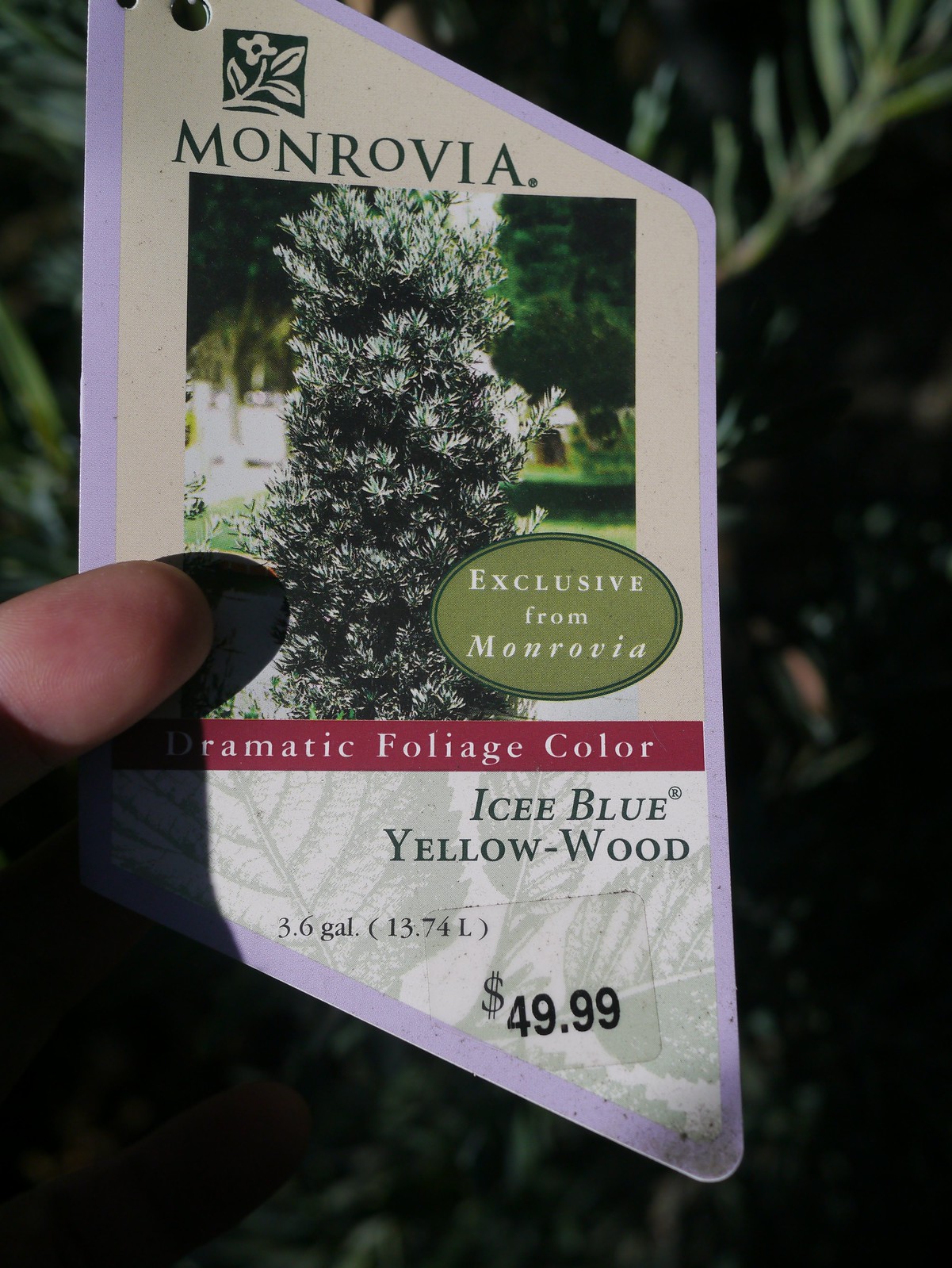A close-up photograph captures a hand holding a nursery tag, originally attached to a tree. The tag, from the reputable brand Monrovia, features their logo and is marked "Exclusive from Monrovia." Prominently displayed is the product name, "Icy Blue Yellowwood," known for its dramatic foliage color. The tag describes the tree's size as 3.6 gallons or 13.74 liters and indicates a price of $49.99. The tag also has a small hole in the upper left for attachment. In the background, partially visible, are the branches of the tree to which the tag was affixed. The label shows a picture of the tree, an oval stating its exclusivity, and a burgundy section highlighting key features. Subtle details like watermark leaves adorn the tag, adding to its visual appeal.